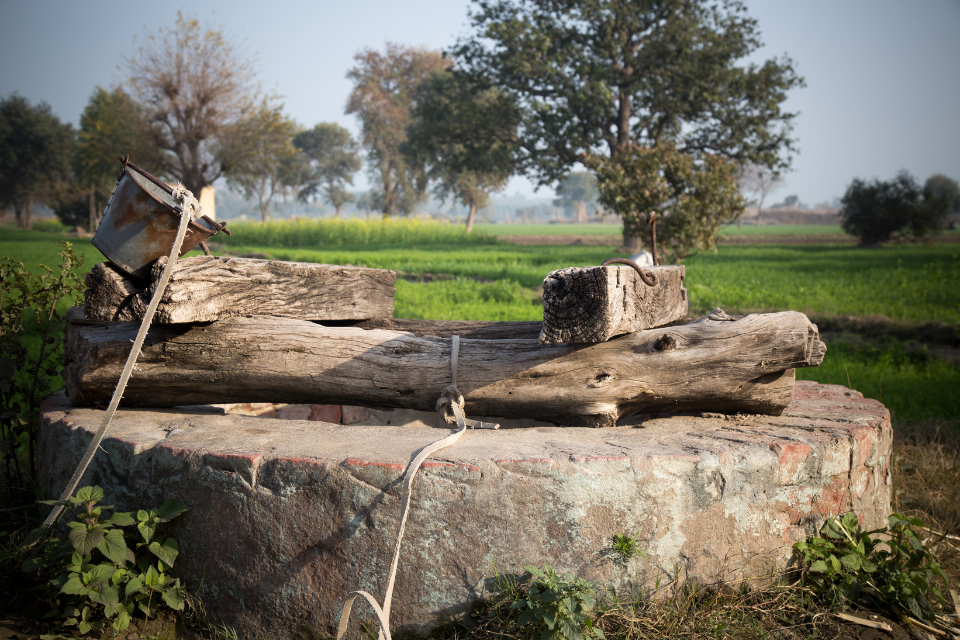The image depicts an outdoor scene dominated by a large, old-style well constructed primarily of thick stone and brick. The well, situated in the foreground, features a horizontal wooden log across its opening, with a rope wrapped around it. Attached to this rope is a rusty bucket, ready to be lowered into the well. Two more logs, resembling railroad ties or four-by-fours, are placed on top of the log, likely to prevent falls. The setting is a vast field with tall grass and a backdrop of sporadically placed large trees. The sky overhead is a moody grayish-blue, heavily clouded, casting a somber tone over the expansive landscape.